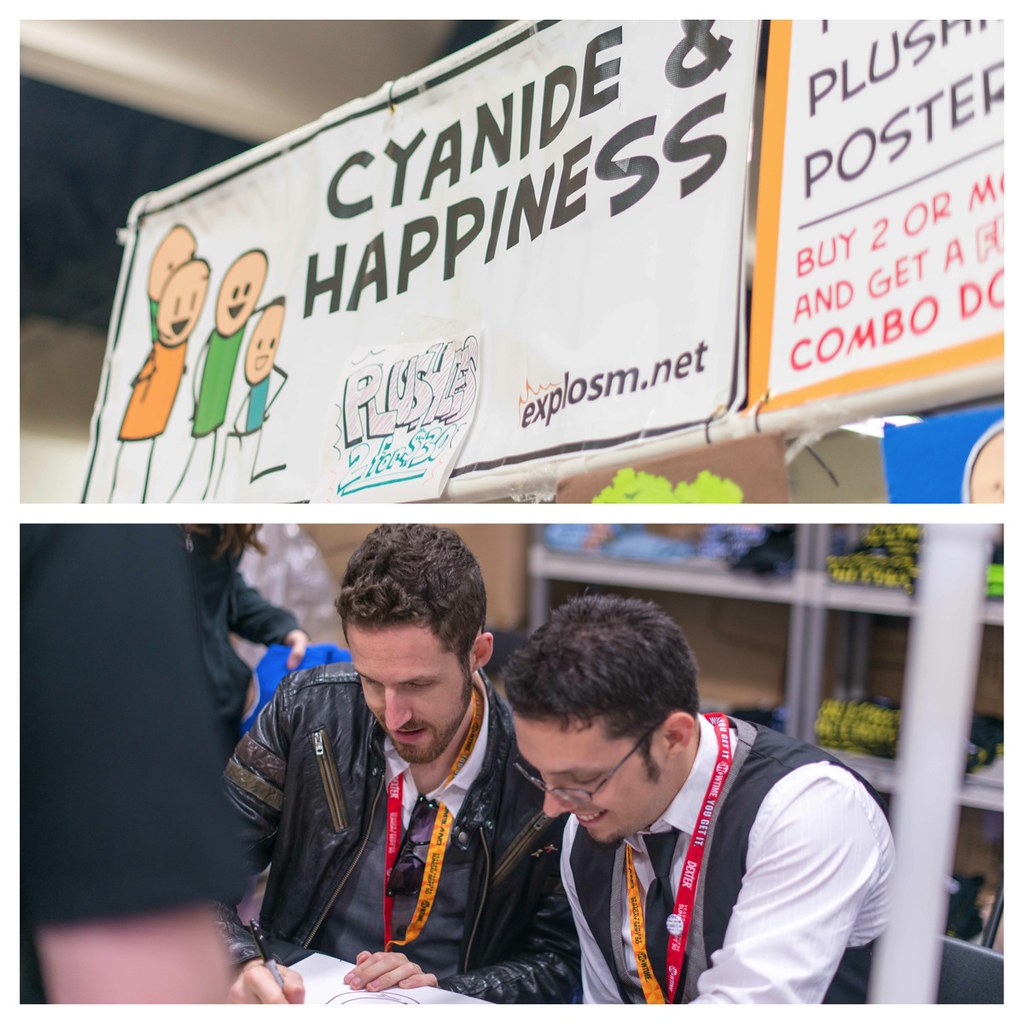The image is split into two panels, with the top panel displaying a colorful and engaging banner for "Cyanide & Happiness," featuring cheerful stick figure characters in orange, green, and blue shirts on a white background. The banner prominently includes the website "explosm.net" and advertises plush toys with a deal of two for $30. There's also a partially visible sign mentioning a special combo offer for purchasing two or more items. The bottom panel captures a scene from what seems to be a Comic Con. It shows two Caucasian men, likely in their late 20s or early 30s, engaged in a book-signing event. Both are wearing convention name tags—one with a tie and the other with a leather jacket and glasses—each holding a Sharpie as they sign autographs for fans. The setting hints at a promotional event, possibly linked with the "Dexter" TV show, as evidenced by the red and gold neck straps one of them is wearing.